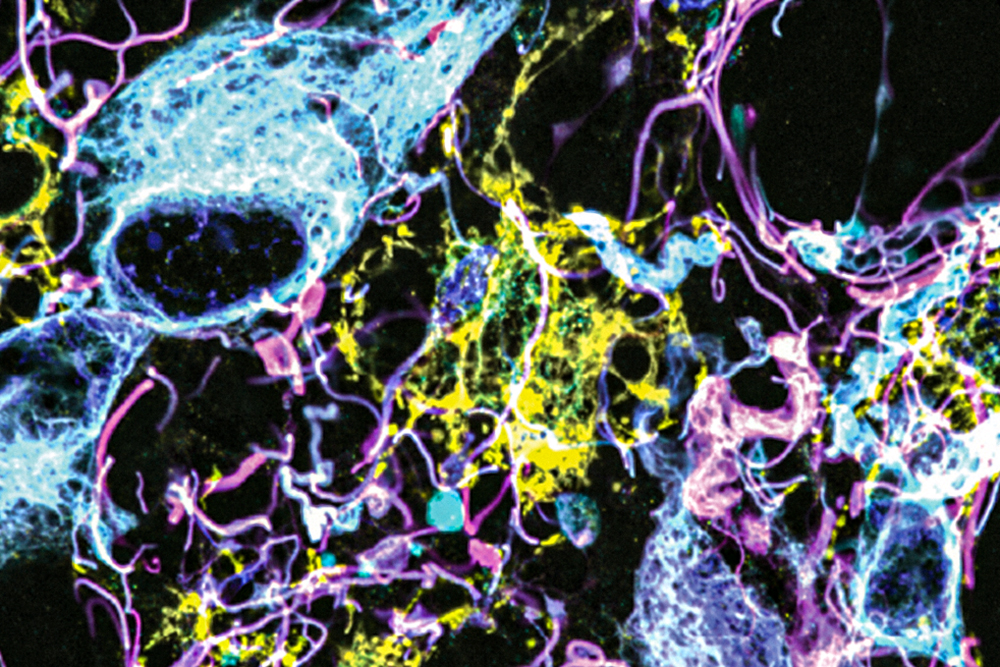The image resembles an abstract art piece, potentially suitable as a desktop background. It features a chaotic yet vibrant mix of neon colors—predominantly light blues, pinks, purples, yellows, and a hint of green—against a stark black backdrop. The yellow color stands out prominently in the center, dominating the composition. The colors are arranged in a manner reminiscent of a splatter painting, with certain elements forming tendril-like, noodle-shaped patterns that seem to be laid out haphazardly. Additionally, there are stringy, cobweb-like, and mesh-netting textures interspersed throughout, creating an intricate, almost scientific appearance. Bright white squiggly lines add a glowing effect, enhancing the image's dynamic and disorganized nature.